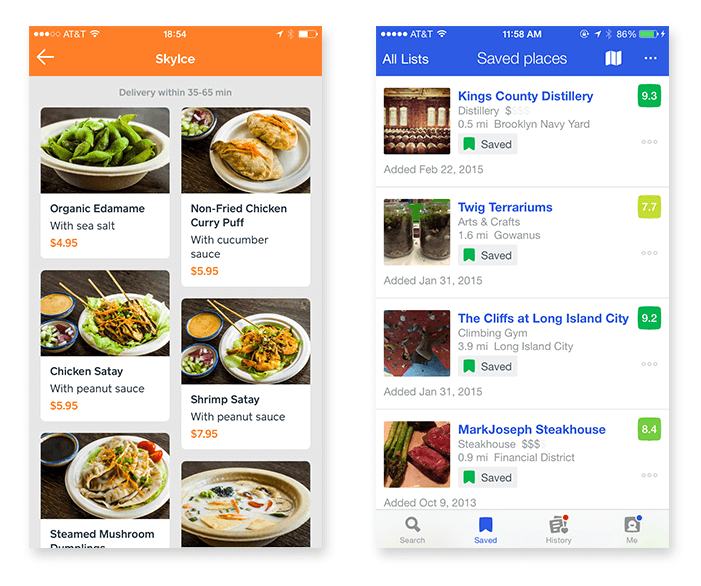The image showcases two smartphone screenshots side by side, displaying distinct content. 

On the left, the AT&T phone screen is marked by an orange status bar at the top, showing the time as 18:54 (or 6:54 PM) with a battery life hovering around 50%. It features an app named "Sky Ice" detailing various food delivery options that promise to arrive within 30 to 65 minutes. The menu items are illustrated with accompanying photos, offering choices like Organic Edamame with Sea Salt for $4.95, Non-Fried Chicken Curry Puff with Cucumber Sauce for $5.95, Chicken Sauté with Peanut Sauce for $5.95, Shrimp Sauté with Peanut Sauce for $7.95, and Steamed Mushroom Dumplings. There is also another dish that is unclear due to the image quality.

On the right, another phone screen with a blue status bar shows the time as 11:58 AM with an 86% battery life, featuring a "Saved Places" list. This list includes King's County Distillery with a rating of 9.3, Twig Terrarium at 7.7, The Cliffs at Long Island City with a 9.2 rating, and Mark Joseph's Steakhouse at 8.4. Each location is accompanied by photos as you scroll down, catering to someone exploring dining and recreational options.